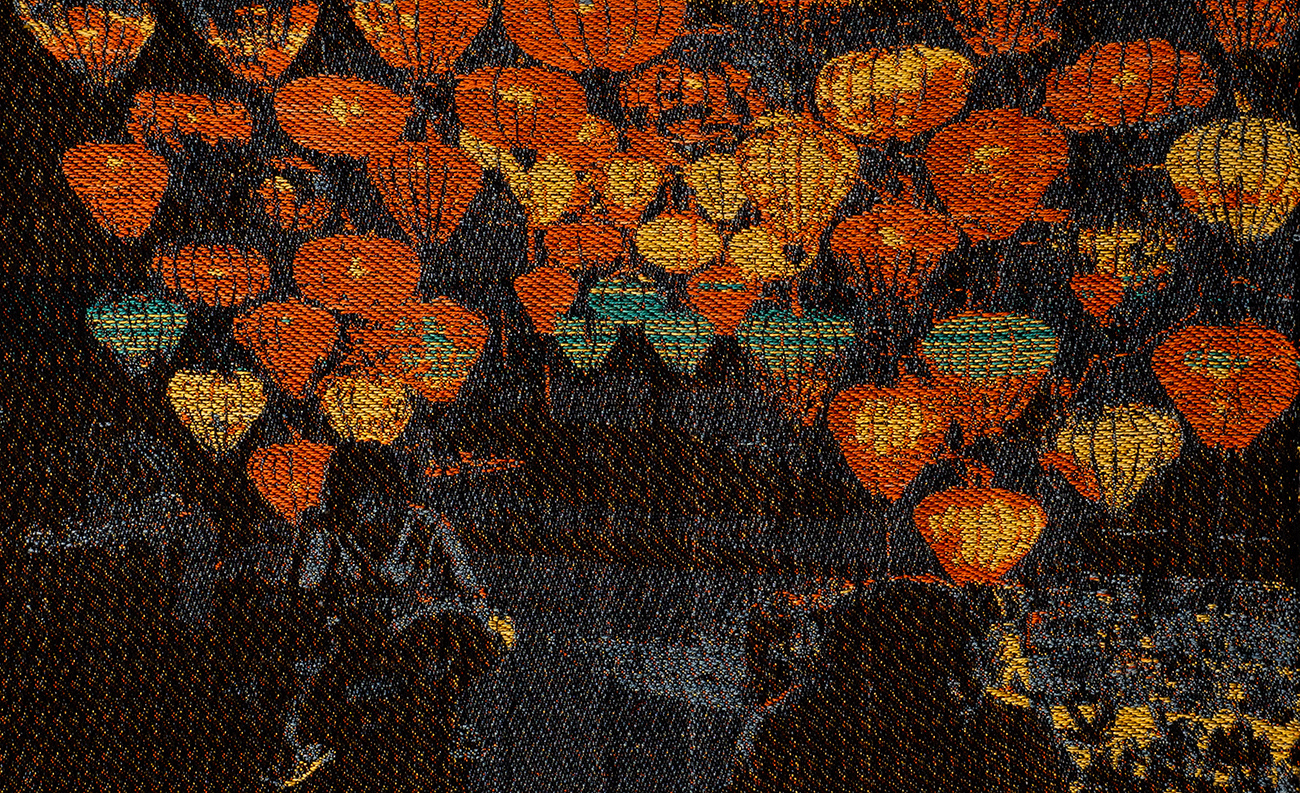The image resembles a knitted pattern depicting a lantern festival. In the dark evening sky, an array of vibrant Chinese lanterns—predominantly red, yellow, and orange with hints of blue and green—float upward. These lanterns, evocative of hot air balloons but with a pumpkin-like look, are densely packed and emit a soft, glowing light. Toward the bottom of the picture, partially obscured by shadows and dark colors, are indistinct figures, possibly people who have released these lanterns. Two figures sit in the foreground, facing away from the lanterns, with one person clearly visible, hands resting in their lap. On the left and right edges of the image, there are faint outlines of houses, blending into the textured, almost fabric-like quality of the scene.